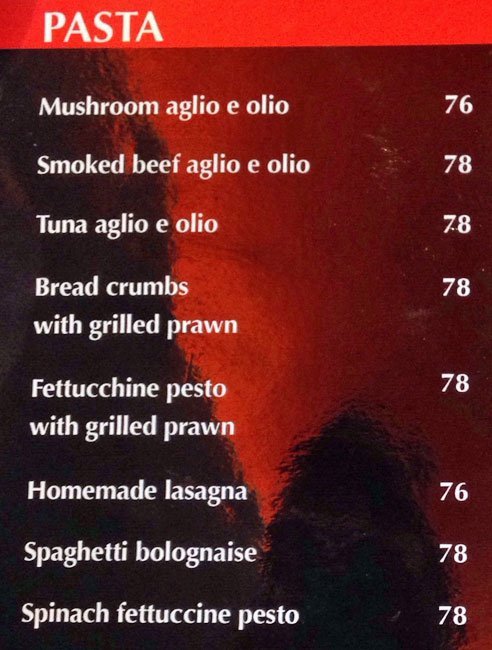The image is a vertically cropped photograph, likely taken on a smartphone, displaying a portion of a menu, possibly from an Italian restaurant. At the very top, there is a red banner with white bold text reading "Pasta." Beneath this, the background transitions to a dark red, almost blood-red metallic color with vertical black sections, creating an indistinct frosted glass effect.

The menu features several pasta dishes listed in white text, some repeating the term "Aglio e Olio." From top to bottom, the dishes and their corresponding prices are:
1. Mushroom Aglio e Olio - 76
2. Smoked Beef Aglio e Olio - 78
3. Tuna Aglio e Olio - 78
4. Breadcrumbs with Grilled Prawn - 78
5. Fettuccine Pesto with Grilled Prawn - 78
6. Homemade Lasagna - 76
7. Spaghetti Bolognese - 78
8. Spinach Fettuccine Pesto - 78

The numbers indicating the prices are aligned on the far right side of the image, also in white text. The background's mixed red and black, frosted glass appearance may obscure finer details, yet the overall theme and pricing are clearly legible. Additionally, there is a faint reflection of the person taking the photograph visible in the background.